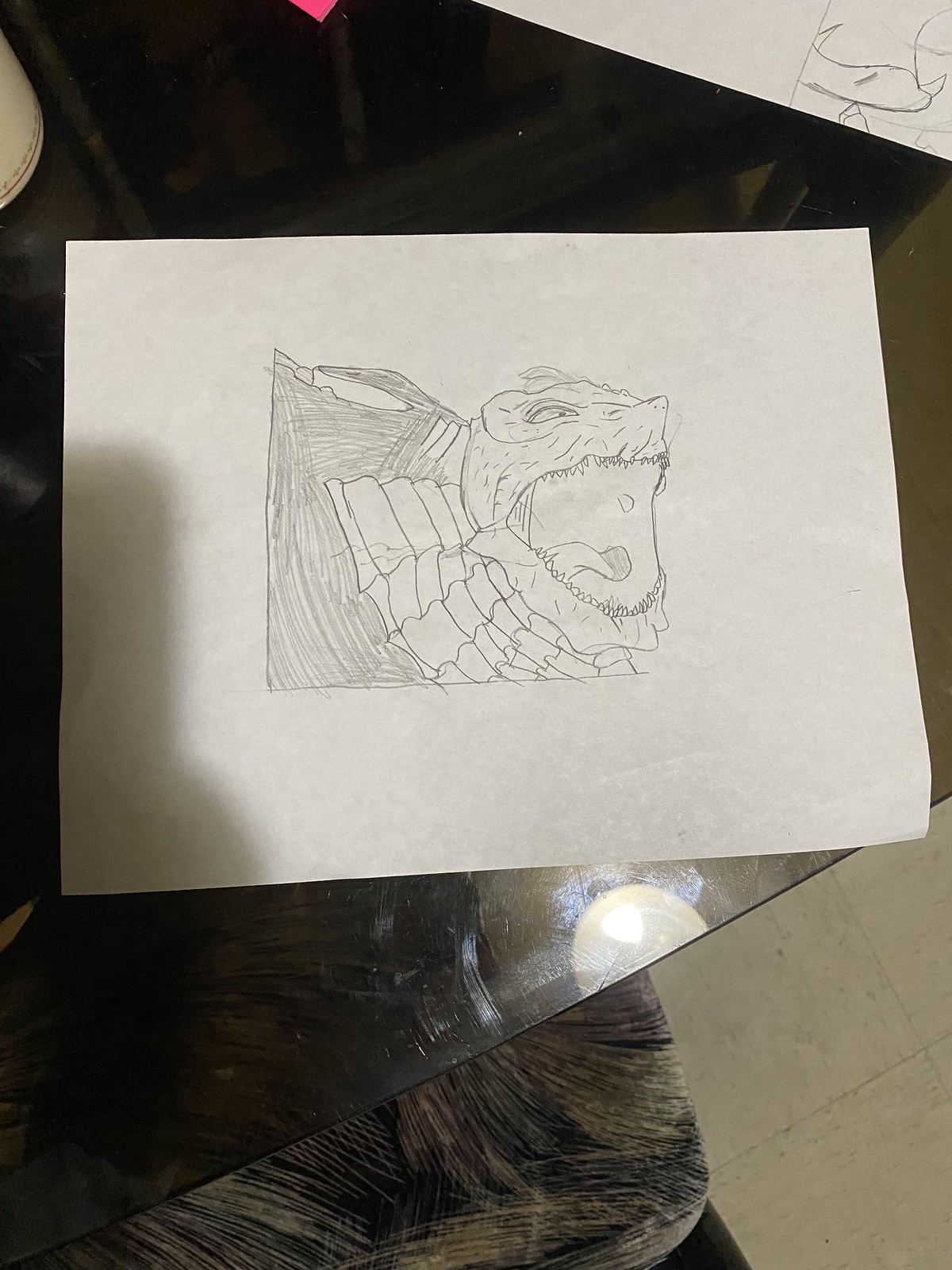A detailed pencil sketch of a lizard-like creature fills the center of a white piece of paper. The creature's mouth is open, revealing a tongue, and its chest is adorned with intricate scales. The back of the creature features darker shading, adding depth to the drawing. A hand-drawn box frames the creature, isolating it on the otherwise blank paper. The paper rests on a glass tabletop, through which the floor beneath is visible. The floor appears to be white tile with subtle brown flecks.